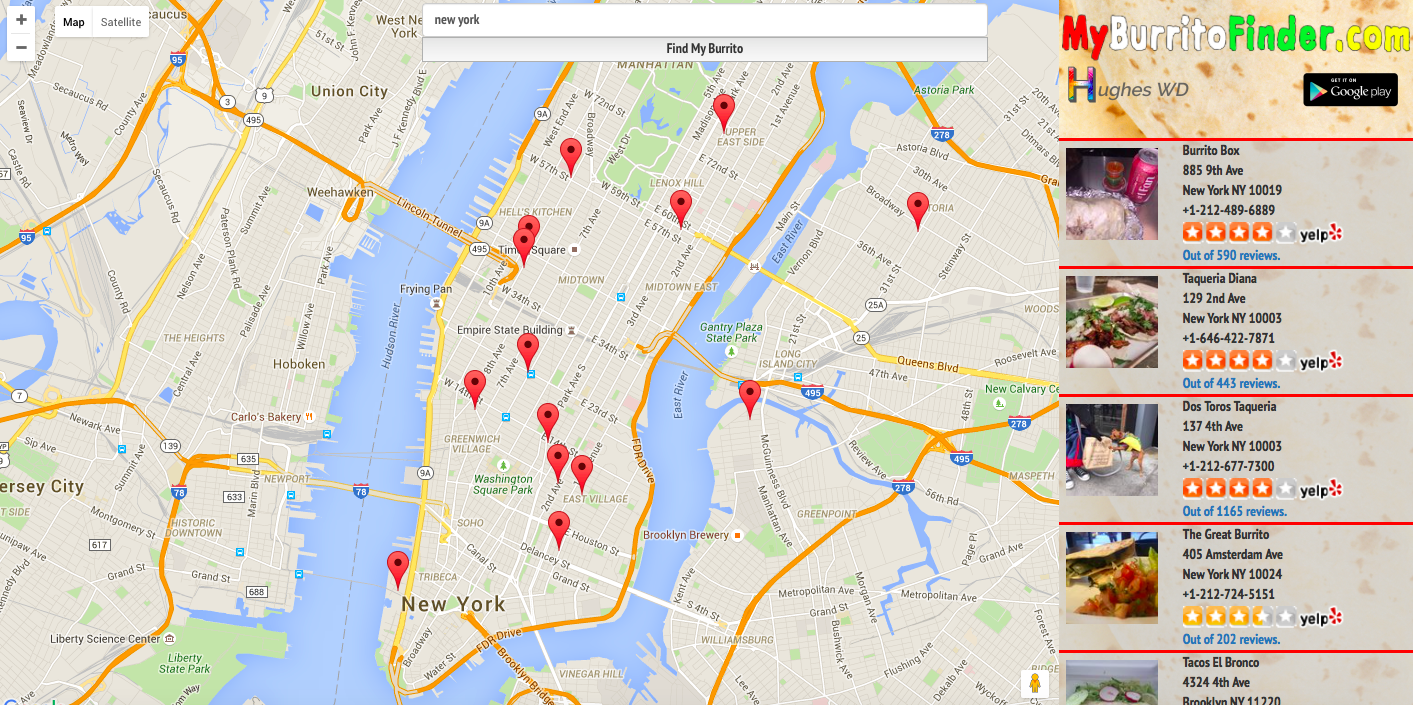This screenshot features the MyBurritoFinder.com website, highlighting its functionality and user interface. The focal point of the image is a map interface that visually represents the area being searched—in this instance, New York. At the top of the webpage is a search bar where users can input the name of a city and a conspicuous button labeled "Find My Burrito" to initiate the search.

On the right-hand side of the screenshot, a sidebar displays a list of burrito establishments in the specified area, each entry complete with a wealth of information: the name of the establishment, its location, phone number, review links, and Yelp links. The visible listings include Burrito Box, Taqueria Diana, Dos Torres Taqueria, The Great Burrito, and Tacos El Bronco. Numerous pinpoints indicating additional burrito spots dot the map, suggesting more results accessible by scrolling.

In the upper left corner of the map, there are controls for zooming in and out, as well as options to toggle between map and satellite views. Overall, this image provides a comprehensive look at how users can utilize MyBurritoFinder.com to locate and research various burrito spots within a chosen city.